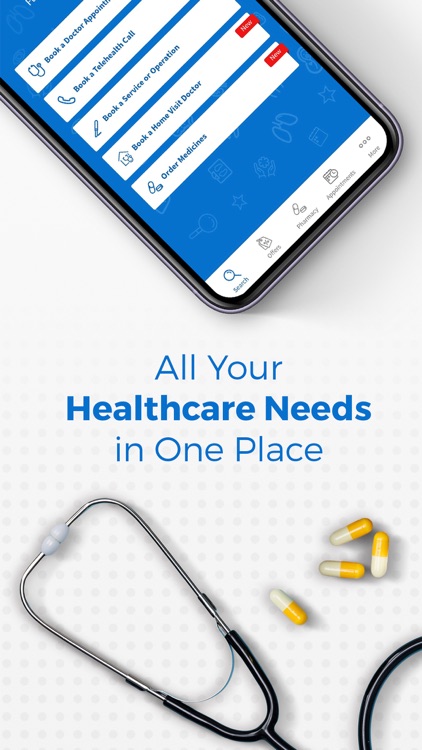This image showcases two medical items arranged on a white background, resembling an advertisement. The photo is taken from a top-down perspective. Centrally positioned text between the two items reads, "All your health care needs in one place."

At the bottom of the image, angled upwards from the right corner, is a part of a stethoscope. The visible section includes the earpiece, extending towards the left, with a small portion of its tubing also visible in the lower right. Adjacent to the stethoscope are four capsule pills, colored yellow and white, neatly lined up.

Towards the top left of the image is a smartphone displaying a medical application. Prominently featured on the app's interface is a "Book a Doctor" button, indicating an option for scheduling medical appointments.